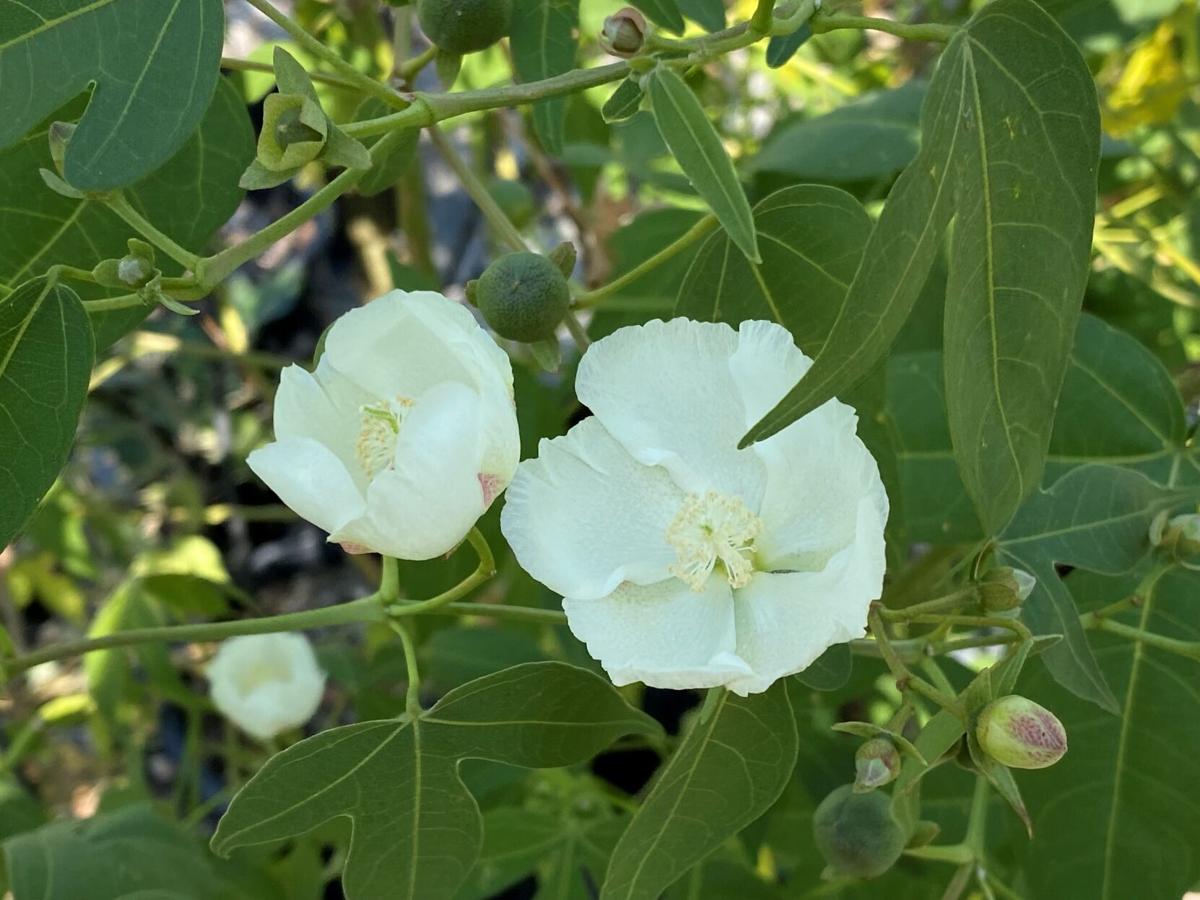This vibrant, sunlit outdoor photo captures a lush green vine adorned with a multitude of leaves and entwining stems. At the center of the image are two striking white flowers in mid-bloom, surrounded by several buds in various stages of opening—ranging from fully closed to partially open. The scene is alive with greenery, punctuated by another blooming white flower in the lower left and additional budding flowers waiting to blossom. The background reveals more leafy plants, all bathed in bright sunlight, enhancing the overall warmth and vitality of the scene. The photo, framed somewhere between a square and a rectangle, immerses the viewer in the intricate beauty of nature with no human presence or text distracting from the floral spectacle.